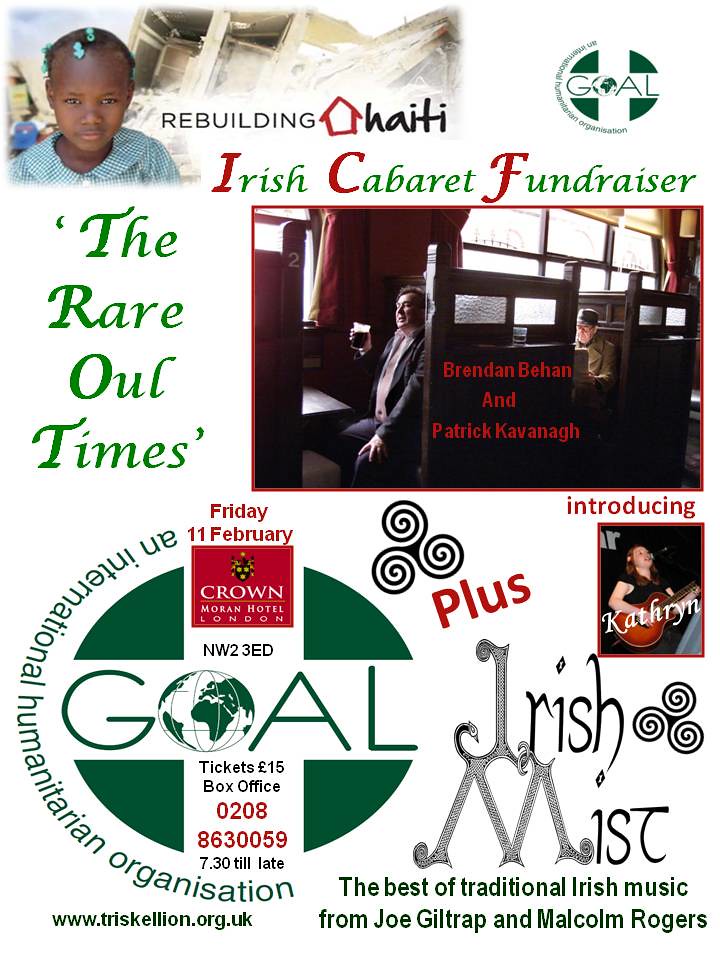This image is a poster promoting a fundraiser event titled "Rebuilding Haiti" and "Irish Cabaret Fundraiser." At the top, it features a photo of a Haitian girl wearing barrettes in her hair and a green and white dress, standing in front of a backdrop of debris or a damaged house. Next to her, the text "Rebuilding Haiti" is displayed, with an outline of a house interposed between the words. Below this, the event title "Irish Cabaret Fundraiser" appears in bold red and green letters. 

On the right side of the poster, a logo for G.O.A.L., an International Humanitarian Organization, is displayed prominently, depicting a green circle with a white cross and a globe encapsulated in the letter 'O'. 

The middle section of the poster features the text "The Rare Old Times" and an image of two men sitting in a pub, one holding a drink, with text labeling them as Brendan Behan and Patrick Kavanaugh/Cavanagh. 

Towards the bottom, additional event details are provided, including ticket information priced at £15 and a box office contact number (0288630059730). Prominently, there is also a mention of Irish Mist, highlighting the musical performances by Joe Giltrap and Malcolm Rogers, who are celebrated for playing the best of traditional Irish music.

Overall, the poster is a collage of various images, text, and graphics, effectively promoting a charity event combining elements of Haitian aid and Irish cultural performances.